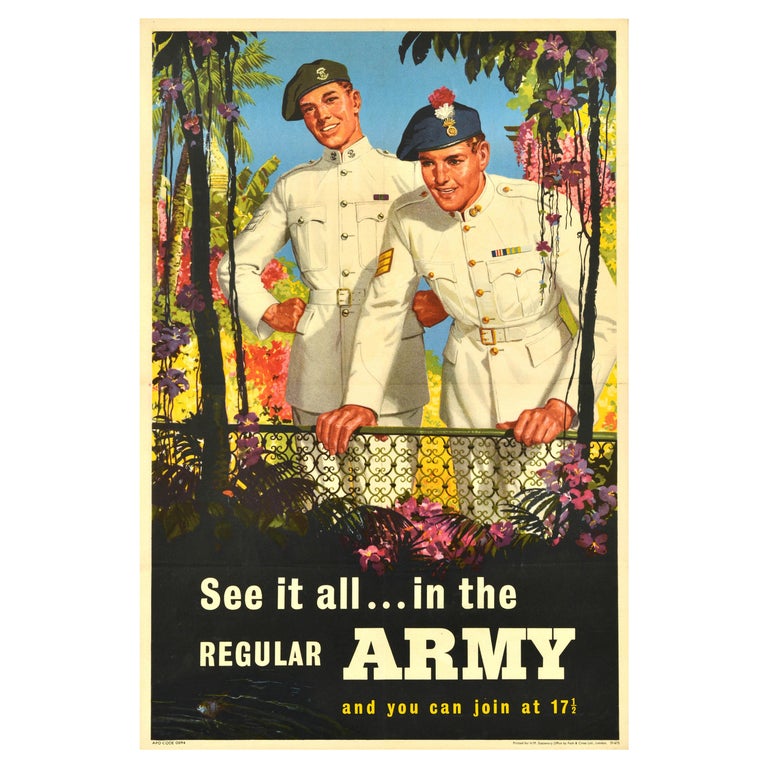This vintage poster, likely from the 1950s, is an illustrated advertisement for the Regular Army, showcasing two soldiers in white dress uniforms. The soldiers, both smiling, are painted against a backdrop of lush tropical foliage, including palm trees and vibrant pink and purple flowers, suggesting an exotic location like Hawaii. One soldier wears a green beret, while the other sports a blue beret adorned with a white and red flower and a medal. One of the men leans over an iron gate, which is adorned with additional colorful flowers, while the other stands confidently with his hands on his hips. The lower portion of the poster features bold white text stating "See it all in the Regular Army," followed by gold text saying "And you can join at 17." The scene aims to portray an inviting, idyllic environment, enticing young individuals to enlist in the Army.